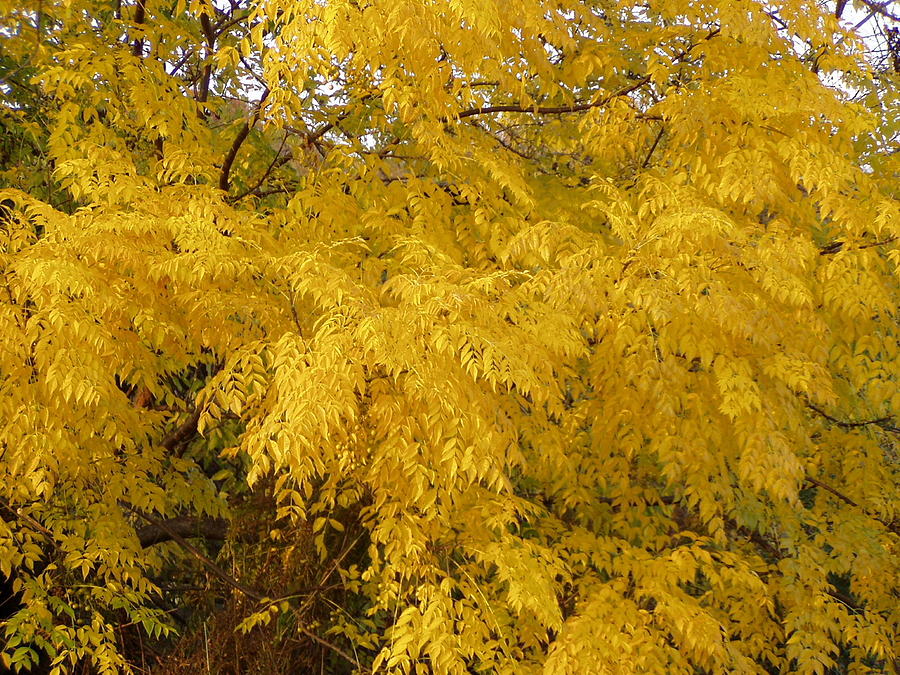The image captures a detailed close-up of tree branches adorned with an array of golden-yellow leaves that dominate the frame. The leaves transition from greenish hues at the lower levels to vibrant yellow further up, indicating a scene set in the fall. The branches extend from the top to the bottom of the image, densely populated with leaves, making the tree trunks less visible. A clear blue sky peeks through the canopy, enhancing the autumnal ambiance and suggesting the photo was taken on a sunny day. The intricate layering of leaves and branches fills the entire composition, emphasizing the richness of the fall foliage.